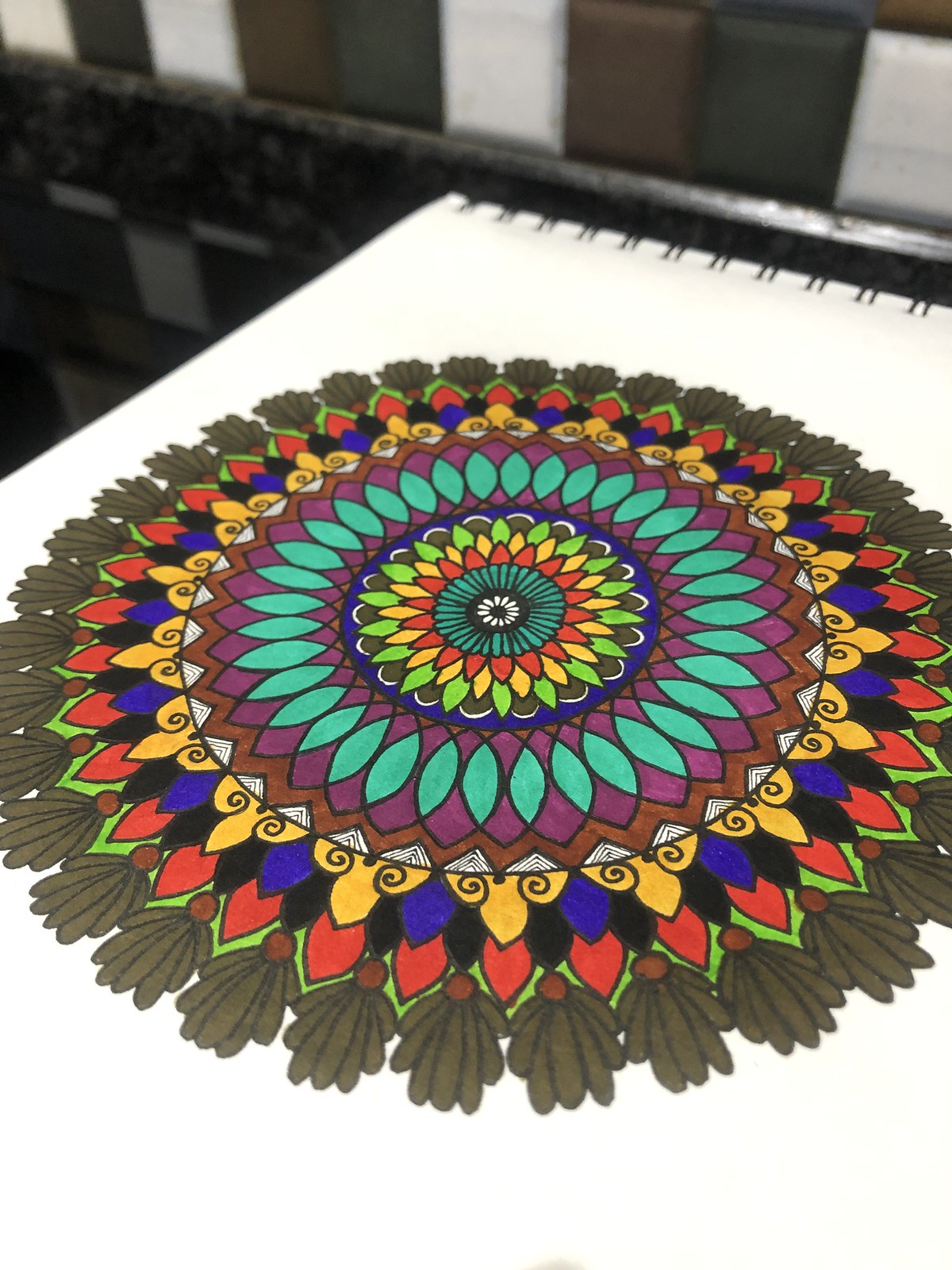A vibrant, multicolored mandala-like illustration adorns a white, ring-bound sketch pad. The pattern, reminiscent of a floral or blossom motif, features a harmonious blend of greens, reds, purples, and browns, with regular, consistent geometric shapes. The intricate design continues with a series of almost leaf-like or tassel shapes in dark olive green along the edges. At its core, the mandala showcases a stark contrast of white and black, surrounded by blue concentric patterns that gradually radiate outward. The background reveals blurred shelves, stocked with additional pads or booklets, contributing to an artistic and creative ambiance.